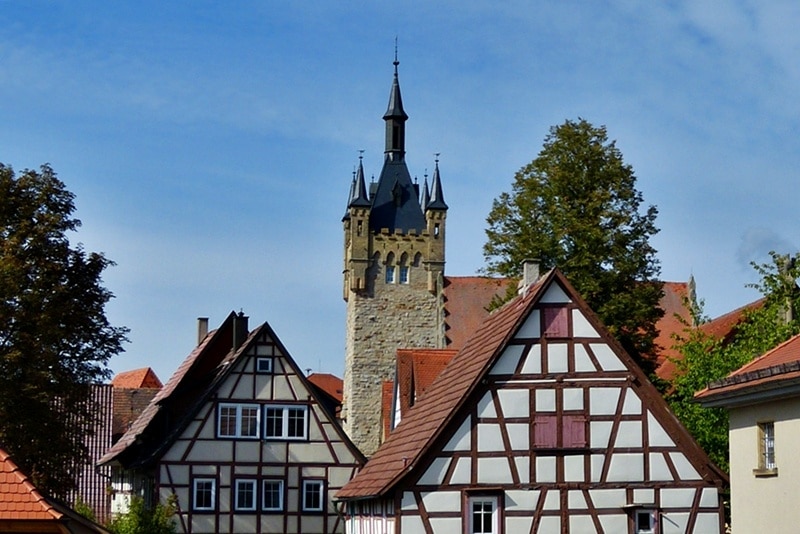This vibrant photograph depicts a picturesque European scene, likely taken in Austria, Germany, or possibly Switzerland or England, on a bright, sunny day in late spring or summer. The foreground is dominated by two distinctive houses with sloped A-frame roofs and unusual patterns on their facades, featuring a mix of white squares, triangles, and other symmetrical shapes, with some parts painted burgundy. The buildings have an appearance of wooden cladding and small windows, giving them a medieval feel. Adjacent to them, there's a third building with a slightly yellowish tinge.

In the background, a grand cathedral with a dark spire towers majestically over the scene. The cathedral features a prominent steeple flanked by four smaller steeples below. A combination of trees adds greenery around the buildings, complementing the scene with their dense, leafy canopies. Most of the upper half of the image is filled with a clear blue sky with a hint of haze. Additionally, various roofs can be seen scattered across the background, enhancing the medieval and European atmosphere of the landscape.